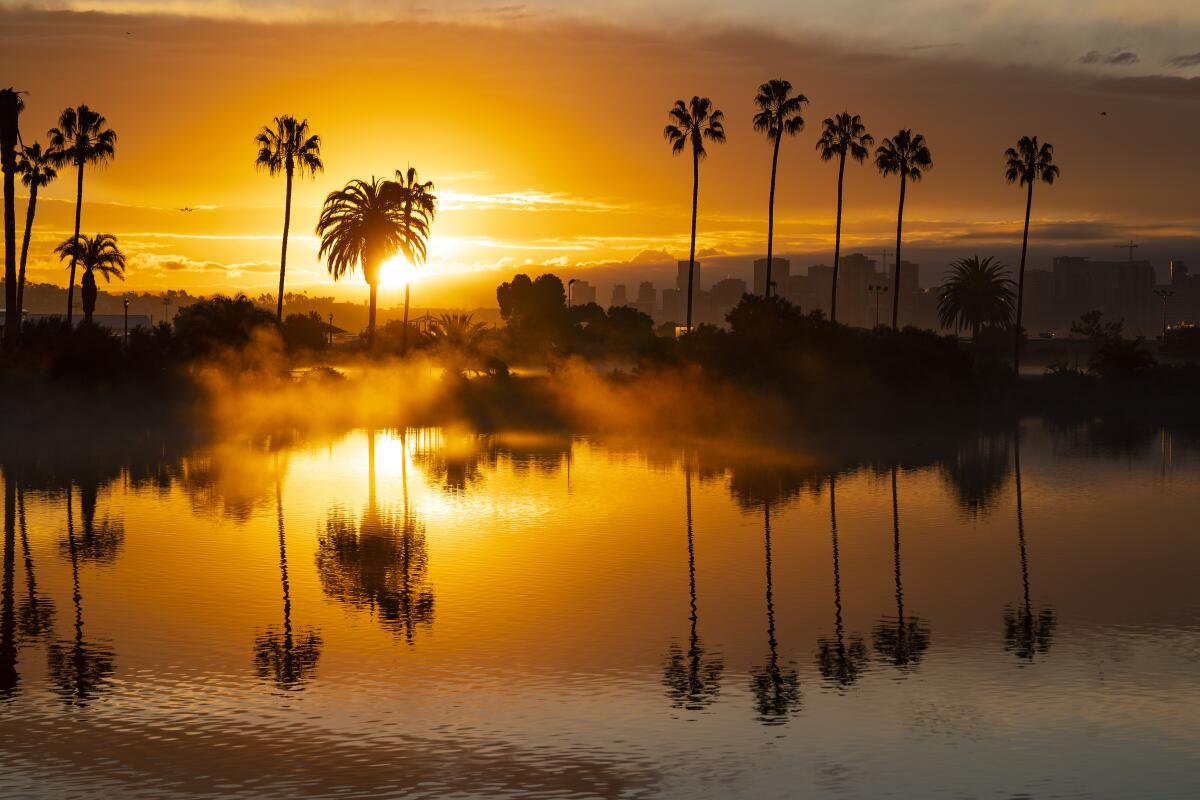This image showcases a striking outdoor scene during either sunrise or sunset, displaying an intense golden-yellow hue that permeates the entire photograph. Captured horizontally, the image features a serene body of water, likely a pond, pool, or lake, situated about 100 feet in front of a line of palm trees. The sun, located low on the horizon, casts a bright, radiant light that creates dramatic silhouettes of the palm trees and high-rise beach condominiums in the background. The sky exhibits a blend of yellow, gray, and hints of black, with subtle white clouds adding to the atmospheric depth. A gentle mist rises from the water, enhancing the tranquility of the moment, while the reflections of the palm trees ripple gracefully across the surface. The entire scene exudes a peaceful, almost artistic quality, capturing the essence of a tranquil moment either at the brink of dawn or the close of day along an ocean or beach setting.